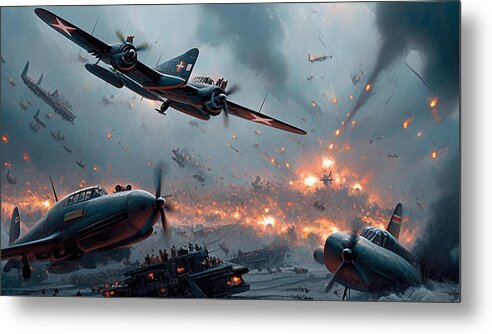The image depicts a chaotic and intense war scene rendered as a poster for a movie or video game. The sky is filled with numerous old-school propeller planes, marked with white X's and a red stripe on their tails, diving down to drop bombs. Many of the planes are engaged in combat, with some being shot down and crashing into the ground. The bottom left of the image shows a crashed plane, along with what appears to be a crew either in a ship or a tank, while another crashed plane is visible in the bottom right with smoke billowing from it. The hazy and snowy gray background is filled with fiery embers and sparks, creating a grim atmosphere as plumes of smoke rise from numerous explosions. The overall scene captures the intensity and chaos of a wartime battle, with planes soaring through the sky and machinery scattered across the snowy battlefield.